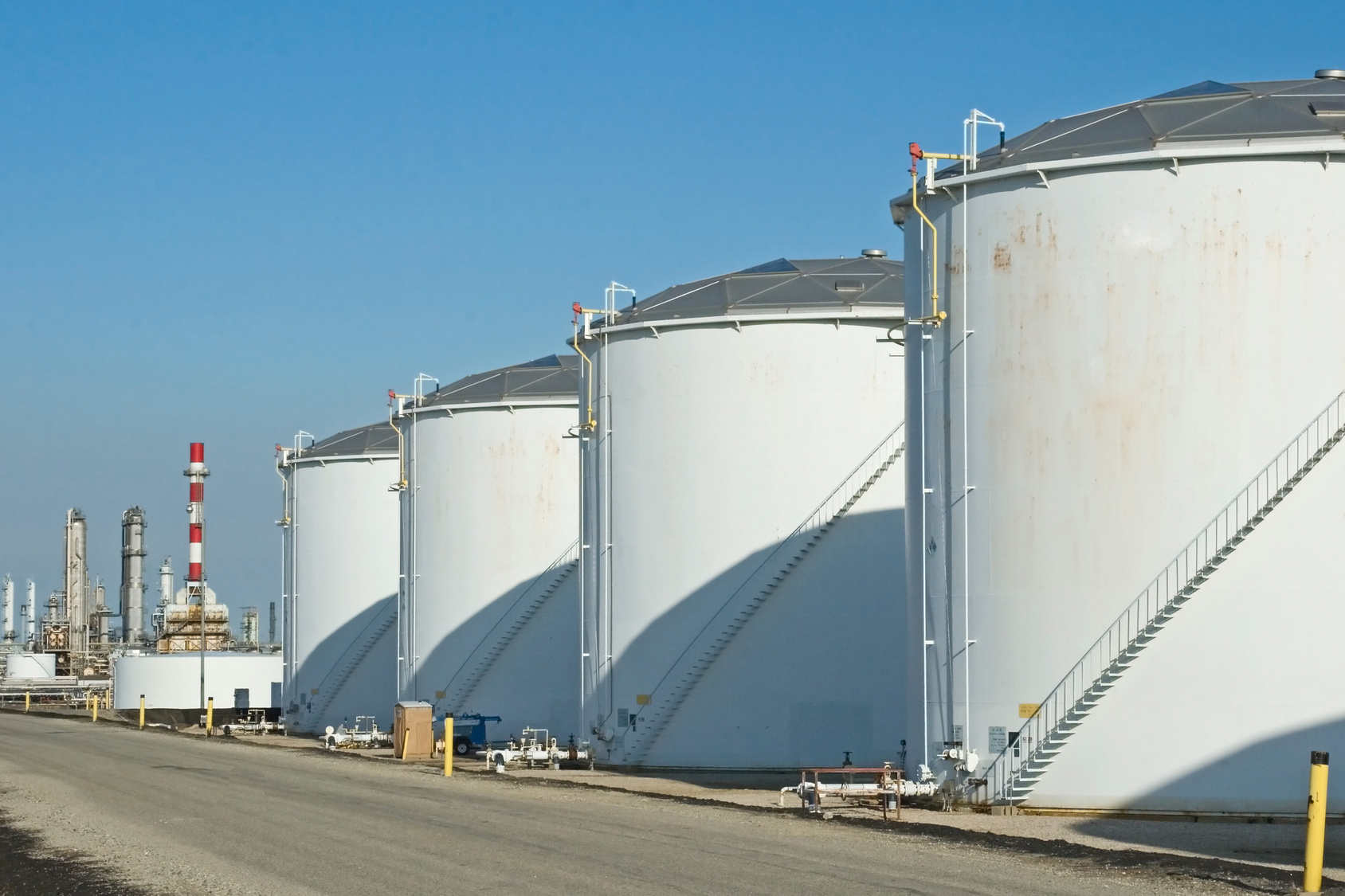The photograph captures four large cylindrical tanks, likely silos, arranged in a neat row in an industrial factory setting. Each silo is predominantly white and equipped with prominent, large staircases. The silos are positioned along a gray gravel road that appears to be part of the facility grounds. In the background, a distinct red and white chimney rises, adding a striking contrast to the scene. The sky is a deep, cloudless blue, suggesting it is daytime with the sun at an angle, contributing to the well-lit ambience. Small figures of people can be seen milling about, accentuating the massive scale of the silos. The overall setting suggests a functional industrial area, possibly for storing materials like water or oil, amidst a well-maintained infrastructure.